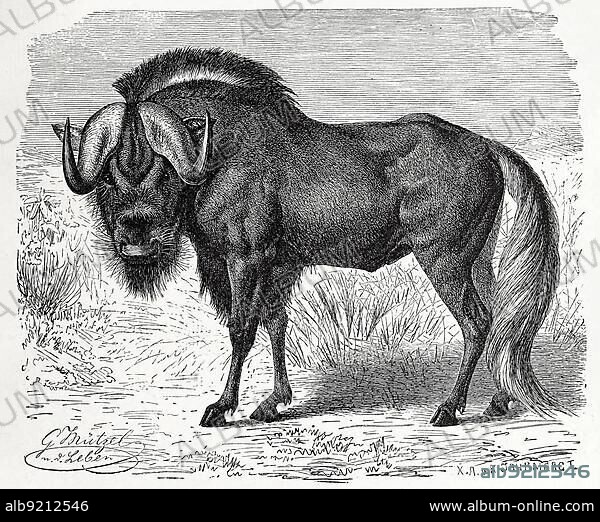This black-and-white hand-drawn illustration depicts a wildebeest, intricately detailed in a medium that resembles black pencil or charcoal. The wildebeest, standing leftward in a grassy field, boasts a muscular body akin to that of a horse. Its distinctive short mane adorns its neck, contrasting with the thick, curved horns that extend from its head, tapering to sharp points. While the drawing overall is predominantly in shades of black, the wildebeest’s tail is rendered slightly lighter. The artwork, which exudes an ancient, almost newspaper-like aesthetic, is accompanied by various markings: In the bottom left corner, names written in cursive – G Mitzel and D Levin – can be found, alongside a numerical watermark reading "ALB 921546." This number is also repeated on the bottom right, beside the text "www.album-online.com." The meticulous detail and the blend of animal traits give the sketch a surreal quality as if it were a mythical creature from a bygone era.